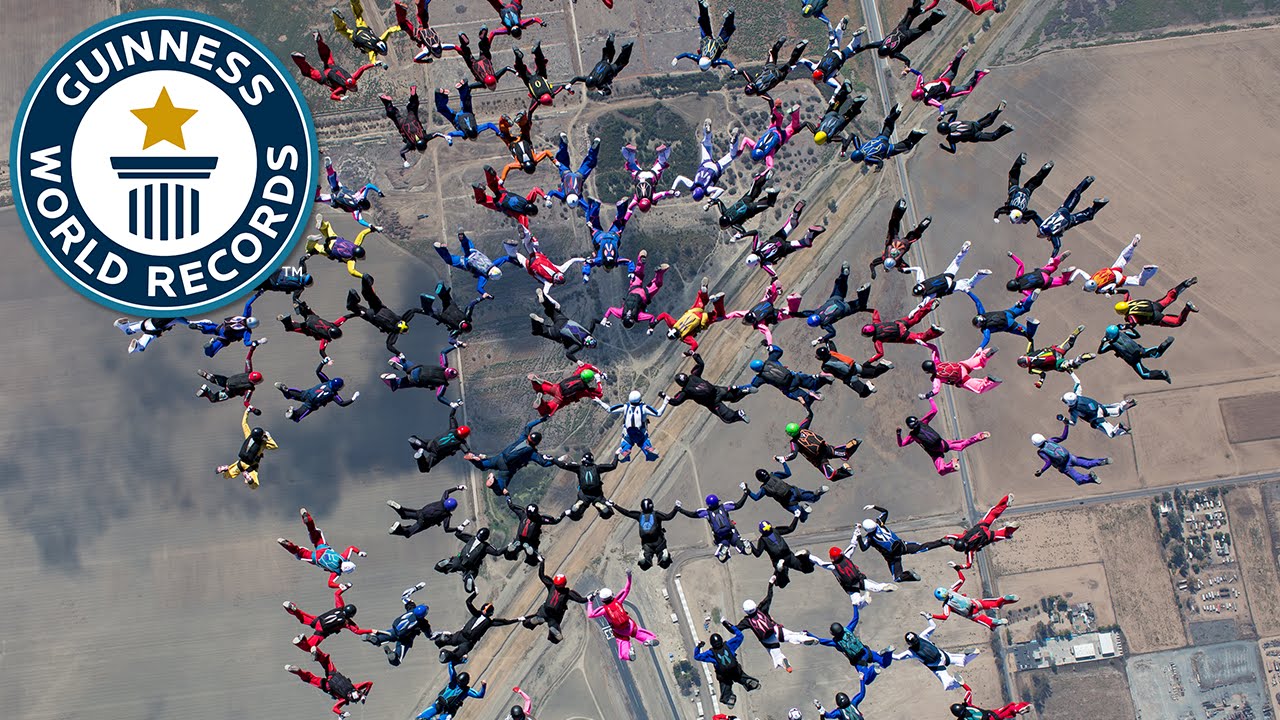This overhead image serves as a YouTube thumbnail for the Guinness World Records channel, depicting an attempted synchronized skydive aiming to break a world record. The top left-hand corner features the Guinness World Records logo, a recognizable medium blue circle with a white pinstripe circle inside and a larger dark blue circle containing the text "Guinness World Records," with a stylized pillar and golden star in the center. The main focus is a large formation of skydivers—estimated to be in the high double digits—dressed in a spectrum of vibrant jumpsuits and parachute packs, ranging from hot pink and purple to red, bright yellow, black, and vibrant blue. At the center of the formation, six divers are connected in a hexagonal shape, with additional skydivers extending outward, holding hands or grabbing the ankles of nearby divers. The background reveals a landscape far below featuring a roadway running diagonally from the bottom left to the top right, surrounded by predominantly gray or brown fields and indistinct structures.